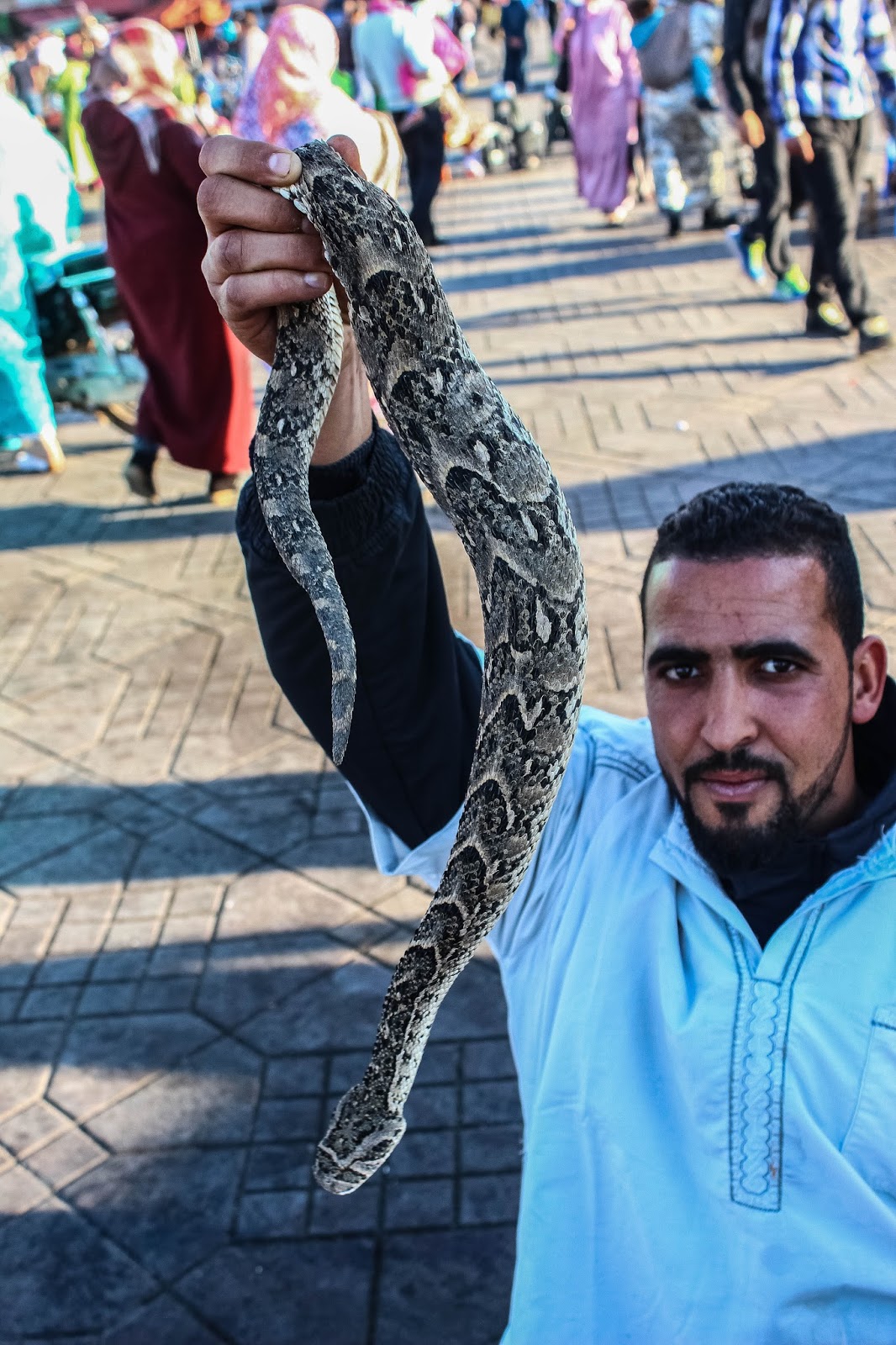In this brightly sunlit outdoor snapshot, a man occupies the bottom right quadrant of the image, extending up to the center and top. He stands on a patterned, abstract pavement shadowed by the intense sunlight behind him, which makes him appear slightly darker than the background. He has short, dark hair and a beard that transitions into a goatee and mustache. He sports a black long-sleeve shirt beneath a casual blue collared shirt featuring a front pattern and a pocket.

The man's right hand holds a medium-sized snake, its back end gripped firmly, with its head facing downward. The snake exhibits a diamondback-like pattern with black and beige scales, and one of its eyes is visible, giving it a menacing appearance. 

Behind the man, a colorful array of people populate the scene, many dressed in vibrant robes and headscarves of purples, blues, and yellows, suggesting a Middle Eastern setting. The pavement beneath him is composed of brown stone pavers, adding to the intricate backdrop of the lively environment.